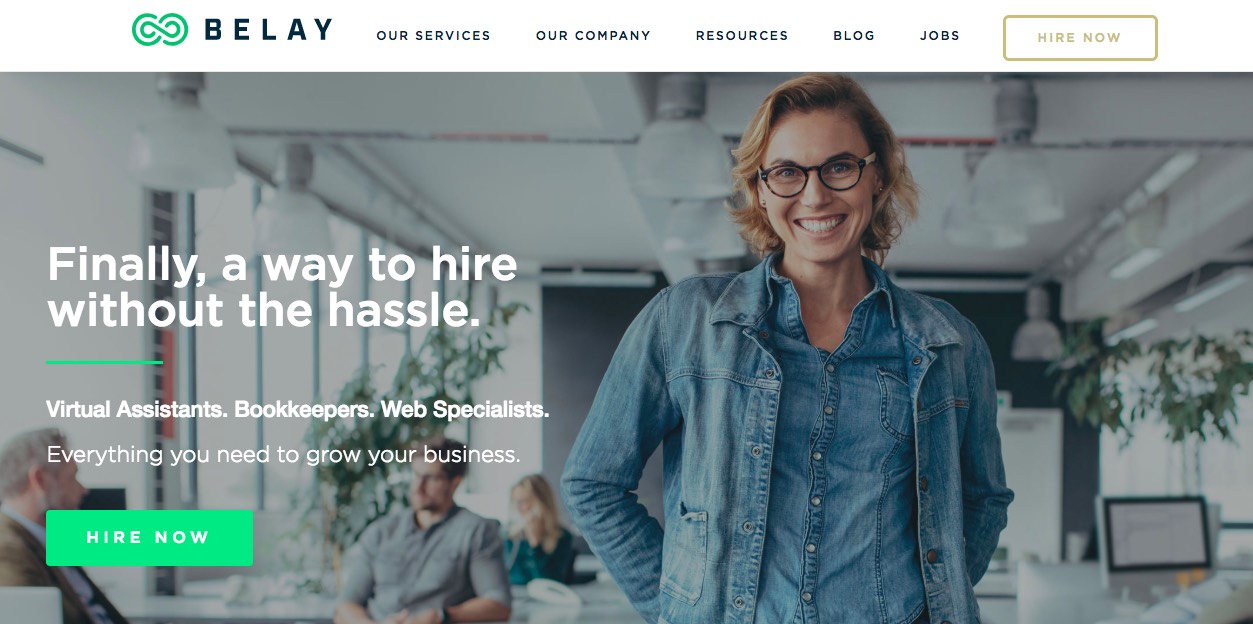The image is a screenshot taken from the Belay website, identifiable by its unique logo in the upper left-hand corner, comprising an infinity symbol integrated into the design. The main navigation menu prominently displays sections titled "Our Services," "Our Company," "Resources," "Blog," and "Jobs," with a conspicuous "Hire Now" button situated at the top of the screen.

At the center of the image, there is a photograph of a woman wearing a jean jacket layered over a denim shirt, exuding a casual yet professional look. Overlaid on her image, in bold white print, is the text: "Finally, a way to hire without the hassle." The promotional text elaborates, listing various services such as virtual assistance, bookkeeping, bookkeepers, and web specialists, indicating that these are essential for enhancing business operations.

In the lower left-hand corner of the image, there's a green button with the label "Hire Now," and just below it, the text "hire you" in a smaller font, emphasizing the call-to-action.